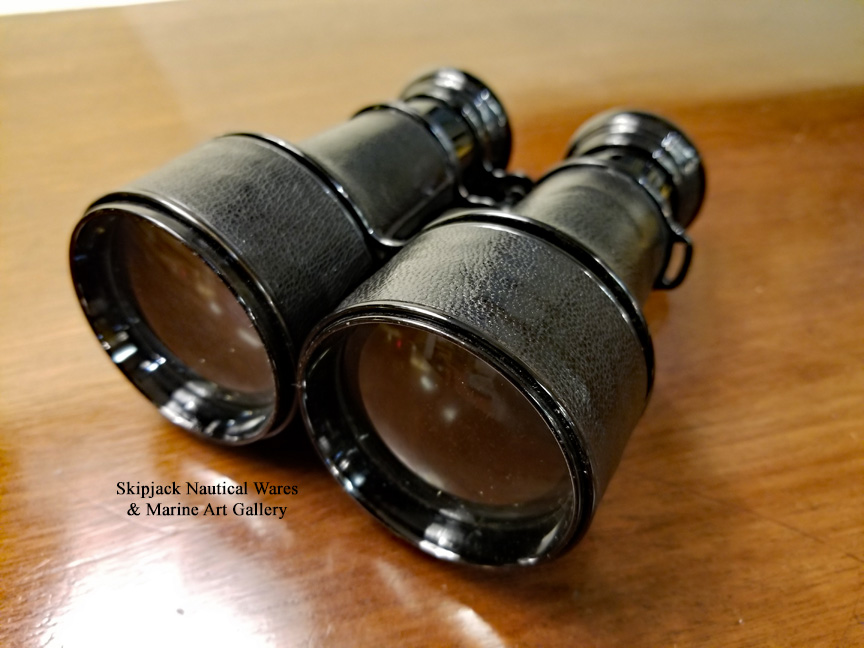A pair of vintage binoculars, primarily black with large objective lenses, is showcased in a close-up shot. The binoculars appear to be made of metal and are potentially wrapped in black suede leather, giving them an antique feel. The image is taken from an angle that highlights the front of the binoculars, with the large lenses facing the viewer. They are resting on a varnished wooden table with a visible light brown grain texture. There's a loop for a neck strap, though the strap itself is not present. In front of the binoculars, there is a sign that reads "Skipjack Nautical Wares and Marine Art Gallery," indicating their nautical background and suggesting they may be more of a decorative art piece rather than purely functional. Light is coming from the bottom left of the image, contrasting with the natural color of the wooden table.